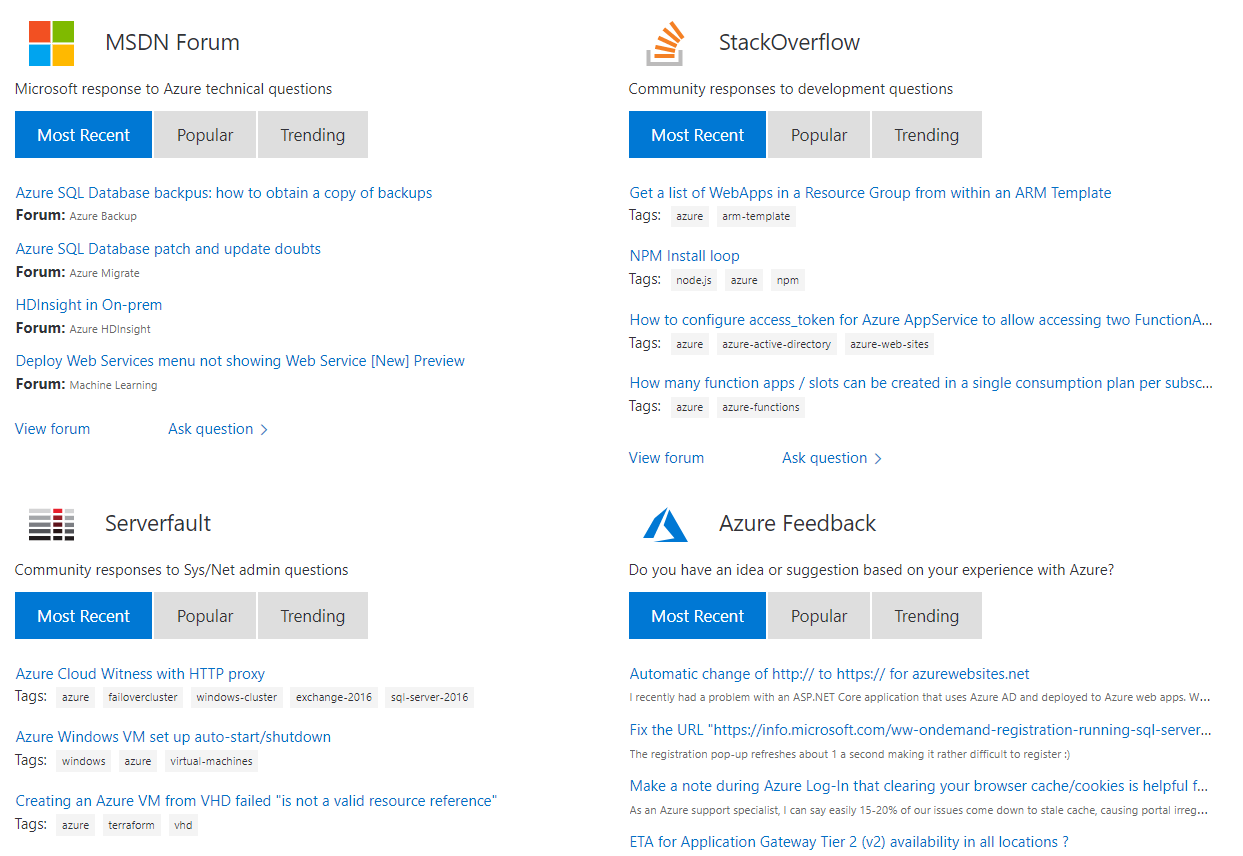**Image Caption:**

The image is divided into four quadrants against a white background, each displaying different forums dedicated to addressing Azure-related queries.

1. **Top Left Quadrant: MSDN Forum**
   - **Logo**: Microsoft logo
   - **Description**: Microsoft response to Azure technical questions
   - **Sorting Options**: Most Recent (selected), Popular, Trending
   - **Topics**:
     - "Azure SQL Database Backup" (Forum: Azure Backup)
     - "How to obtain a copy of backups" (Forum: Azure Backup)
     - "Azure SQL Database Patch and Update doubts" (Forum: Azure Migrate)
     - "HD Insight in on-prem" (Forum: Azure HD Insight)
     - "Deploy web services menu not showing web services (New Preview)" (Forum: Machine Learning)
   - **Buttons**: Visit Forum, Ask a Question

2. **Top Right Quadrant: Stack Overflow**
   - **Logo**: Appears to show orange lines entering a gray "U"
   - **Description**: Community response to development questions
   - **Sorting Options**: Most Recent (selected), Popular, Trending
   - **Topics**:
     - "Get a list of web apps in the resource group from within the ARM template" (Tags: Azure, ARM template)
     - "NPM install loop" (Tags: node.js, Azure, npm)
     - "How to configure access token for Azure app services to allow accessing to function A" (Tags: Azure, Azure Active Directory, Azure websites)
     - "How many function apps/slots can be created in a single consumption plan per subscription" (Tags: Azure, Azure functions)
   - **Buttons**: Visit Forum, Ask a Question

3. **Bottom Left Quadrant: Serverfault**
   - **Logo**: Gray and red design
   - **Description**: Community responses to sys/net admin questions
   - **Sorting Options**: Most Recent (selected), Popular, Trending
   - **Topics**:
     - "Azure Cloud Witness with HTTP proxy" (Tags: Azure failover cluster, Windows cluster, Exchange 2016, SQL Server 2016)
     - "Azure Windows VM setup, auto start/shut down" (Tags: Windows, Azure, virtual machines)
     - "Creating an Azure VM from VHD failed, not a valid resource reference" (Tags: Azure, Terraform, VHD)
   - **Buttons**: (Not visible in the screenshot)

4. **Bottom Right Quadrant: Azure Feedback**
   - **Logo**: Blue triangular logo
   - **Description**: "Do you have an idea or suggestion based on your experience with Azure?"
   - **Sorting Options**: Most Recent (selected), Popular, Trending
   - **Topics**:
     - "Automatic change from HTTP to HTTPS for Azure websites.net" 
     - "Fix the URL issues with Microsoft SQL Server registration"
     - "Advise to clean web browser cache/cookies"
     - "ETA for Application Gateway tier two V2 availability in all locations"

The screenshot serves as a comprehensive view into the various platforms where users can seek, share, and discuss information and issues related to Microsoft's Azure services.